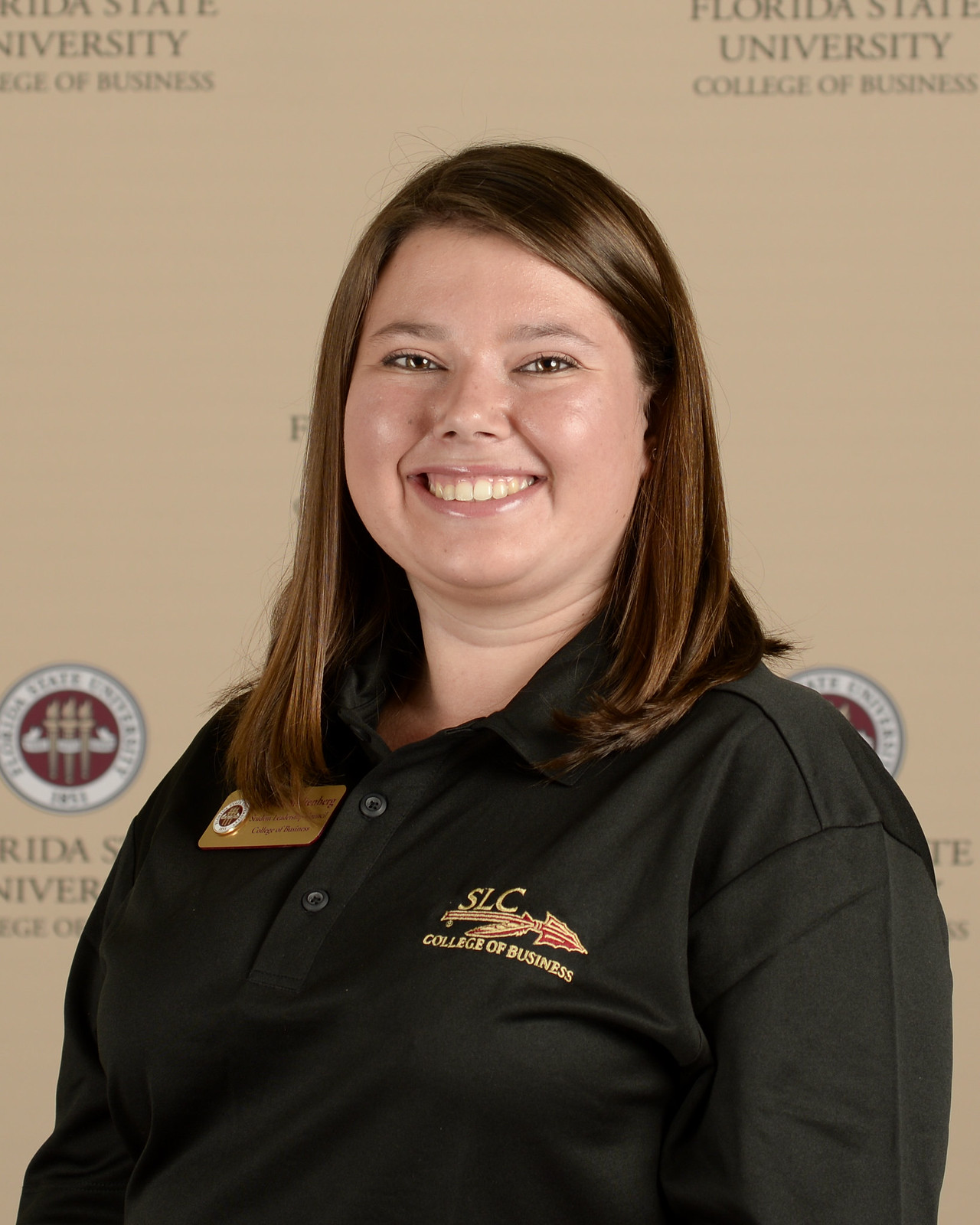This image features a young woman with shoulder-length straight brown hair and possibly hazel eyes, standing or sitting in front of a cream-colored backdrop adorned with the Florida State University College of Business logo. She wears a black polo shirt with two buttons, featuring the SLC College of Business logo on the chest. Additionally, she has a gold, square name tag pinned to the left of the logo, though the text on it is partially obscured by her hair. The woman has a broad, warm smile and appears to be slightly chubby in the face. Behind her, various text and emblems of Florida State University College of Business are visible, including one with a red center and white circular border partially seen over her right shoulder. This setting suggests it might be a faculty or promotional photo for the College of Business.